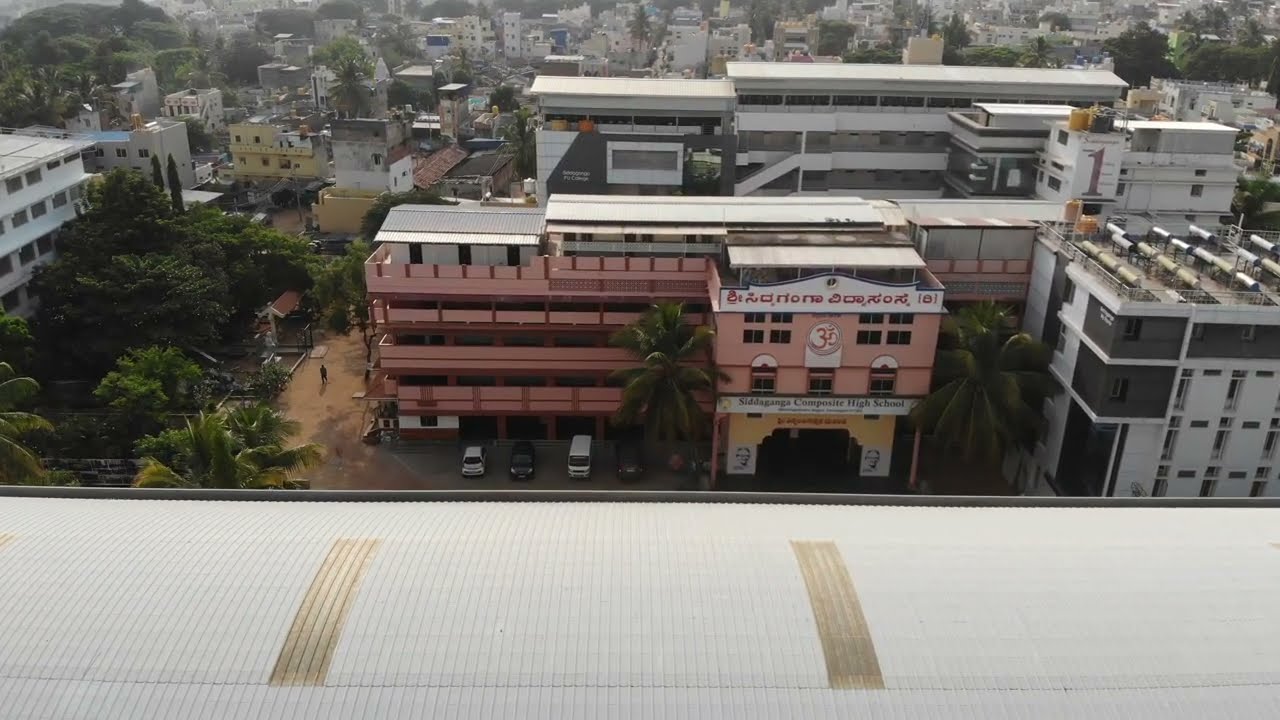In this photograph taken from a rooftop with white shingles, the perspective shows a panoramic view of a diverse urban landscape. Dominating the center of the image is a large, four-story building with a coral pink exterior and a flat roof, featuring a prominent white sign at the top with red lettering in a foreign language. The structure, which has the architectural style of an office or possibly a motel, boasts an arched entrance and has several vehicles, including cars and vans, parked in front. A tall palm tree stands prominently before the building, adding to the tropical aesthetic.

On either side of this central building, there are white apartment buildings rising five to six stories high. To the left of the coral pink building, a lush, expansive patch of tall, tropical trees and palm trees stretches out, providing a verdant contrast to the urban environment. In the background, fading into the distance, are numerous other white apartment buildings interspersed with occasional trees, creating a dense and vibrant skyline against the partly cloudy sky.